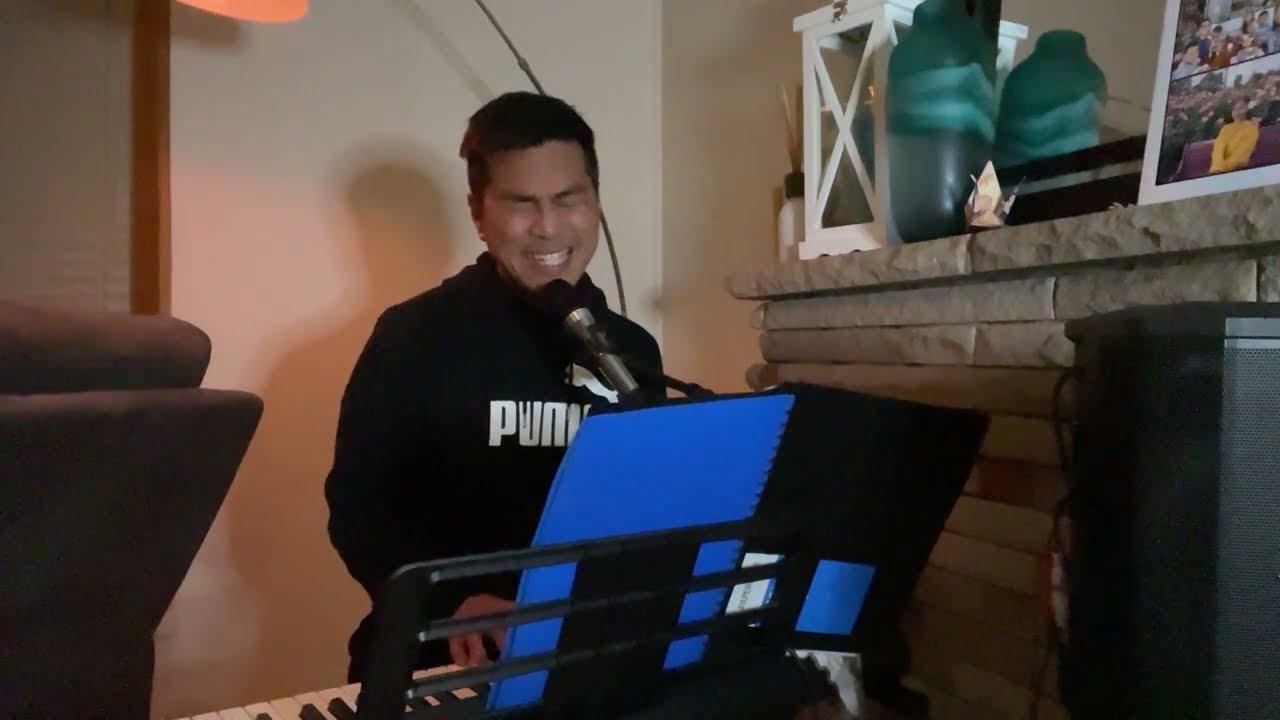In this image, a man is captured in the midst of a heartfelt musical performance in a cozy room. He is seated, playing an electronic keyboard that rests on a stand, with sheets of music placed on it. The music sheets are distinctive with their electric blue and black colors. Engaged deeply in his performance, the man is singing into a microphone, his eyes closed and a smile suggesting his immersion in the music. He sports a black hoodie emblazoned with the Puma logo in white, his short dark hair complementing his casual yet focused demeanor.

The backdrop features a gray stone fireplace mantle adorned with green glass vases, a lit wooden box, and various photographs and artifacts that add a personal touch to the setting. Behind him, his shadow is cast on the wall, hinting at a dimly lit environment with a lamp overhead, though only its top is visible.

To his side, a purple couch or recliner chair is partially visible, adding to the room’s homey feel. A window with blinds and a speaker can also be seen, contributing further to the lived-in ambiance of the space. The overall scene captures a moment of artistic expression amidst a warm, inviting setting.